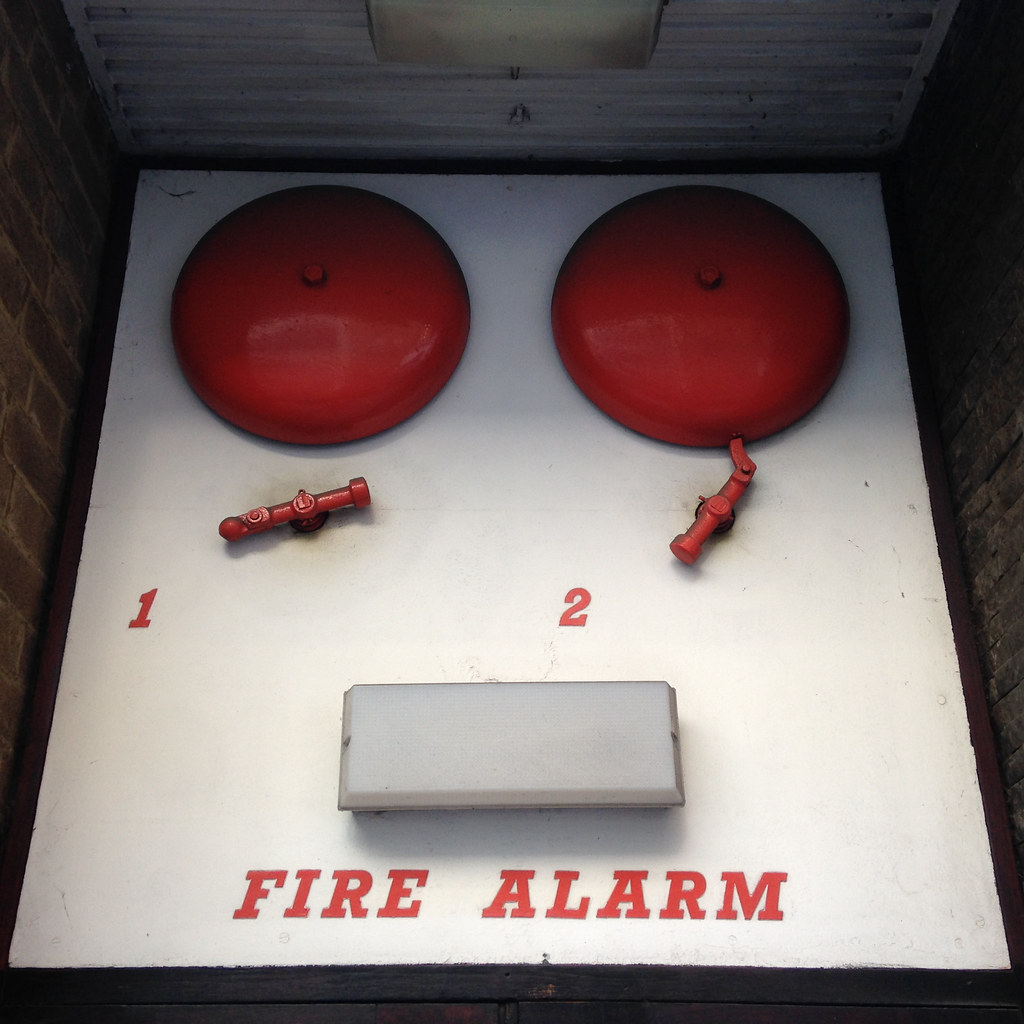This photograph showcases an antiquated fire alarm system set against a white background that is framed by two brick walls. The top portion of the image is engulfed in shadows while the bottom part remains well-lit. At the top, two round, red metal half-circles—reminiscent of old-school bells—are focal points. These bells, numbered '1' on the left and '2' on the right in red, have corresponding levers below, although one lever appears dysfunctional, suggesting it might not activate the bell properly. Directly beneath the bells is a white rectangular box that could serve as a light indicator when the alarm is triggered. Below this box, the phrase "FIRE ALARM" is stenciled in a retro font, painted in striking red. A dark wood border runs along the bottom part of the fire alarm setup, adding a rustic touch to this vintage safety apparatus.